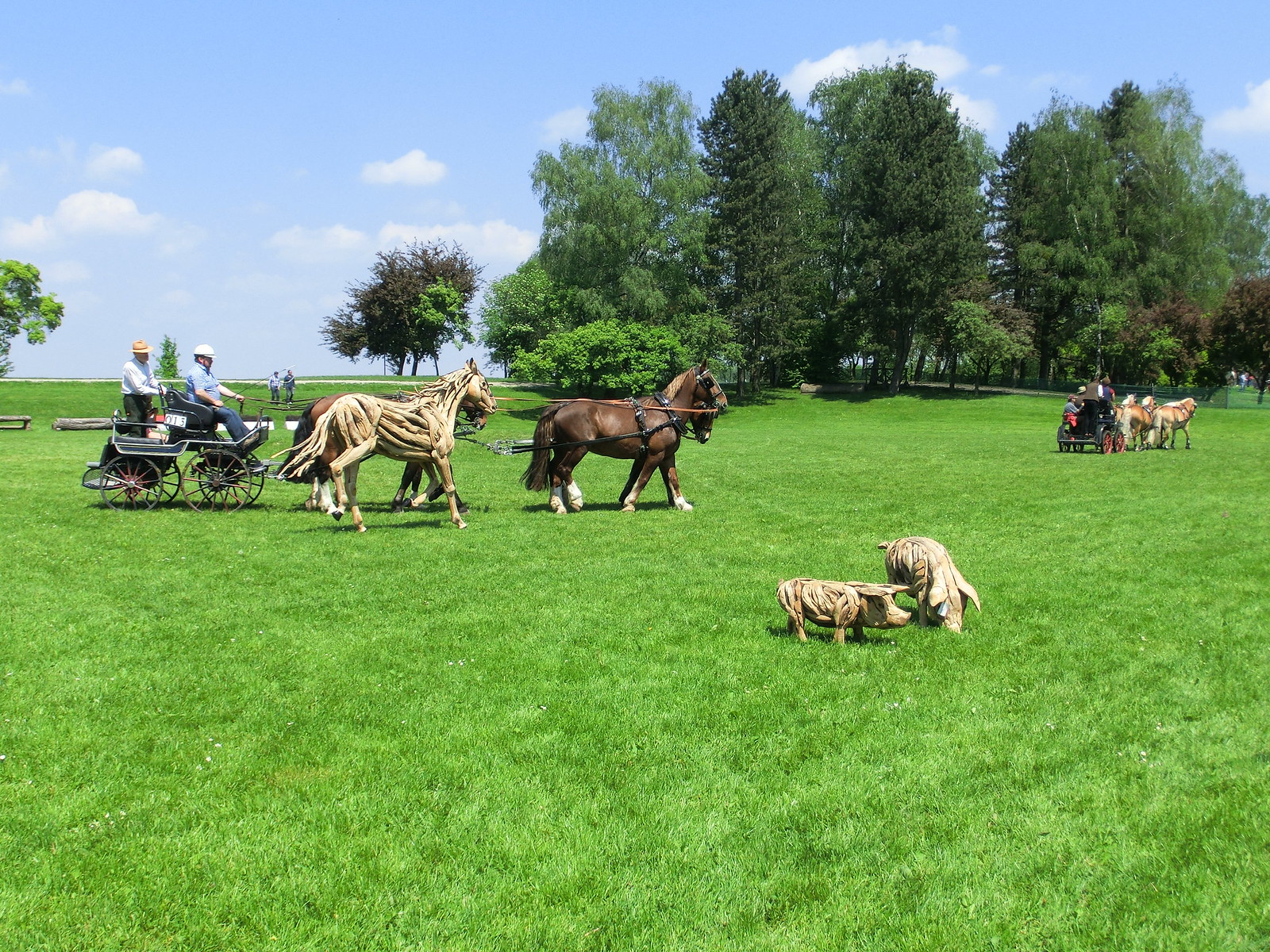The photograph depicts an outdoor scene in a well-maintained green field, surrounded by trees with lush green leaves. In the foreground, two wooden pig sculptures are positioned to the right. To the left, there is a horse-drawn carriage occupied by two men dressed in blue shirts and brimmed hats. This carriage is pulled by a combination of real and wooden horses, with a prominent brown live horse central to the image, and another horse, possibly a tan one, tethered behind it. The wooden horse displays meticulous craftsmanship, mimicking equine musculature with its carved wooden pieces. Further back, a second carriage with red wheels can be seen, featuring horses that appear to be pulling it as well. This distant carriage blends into the expansive grassy landscape, which is framed on the right side and in the background by a variety of trees.